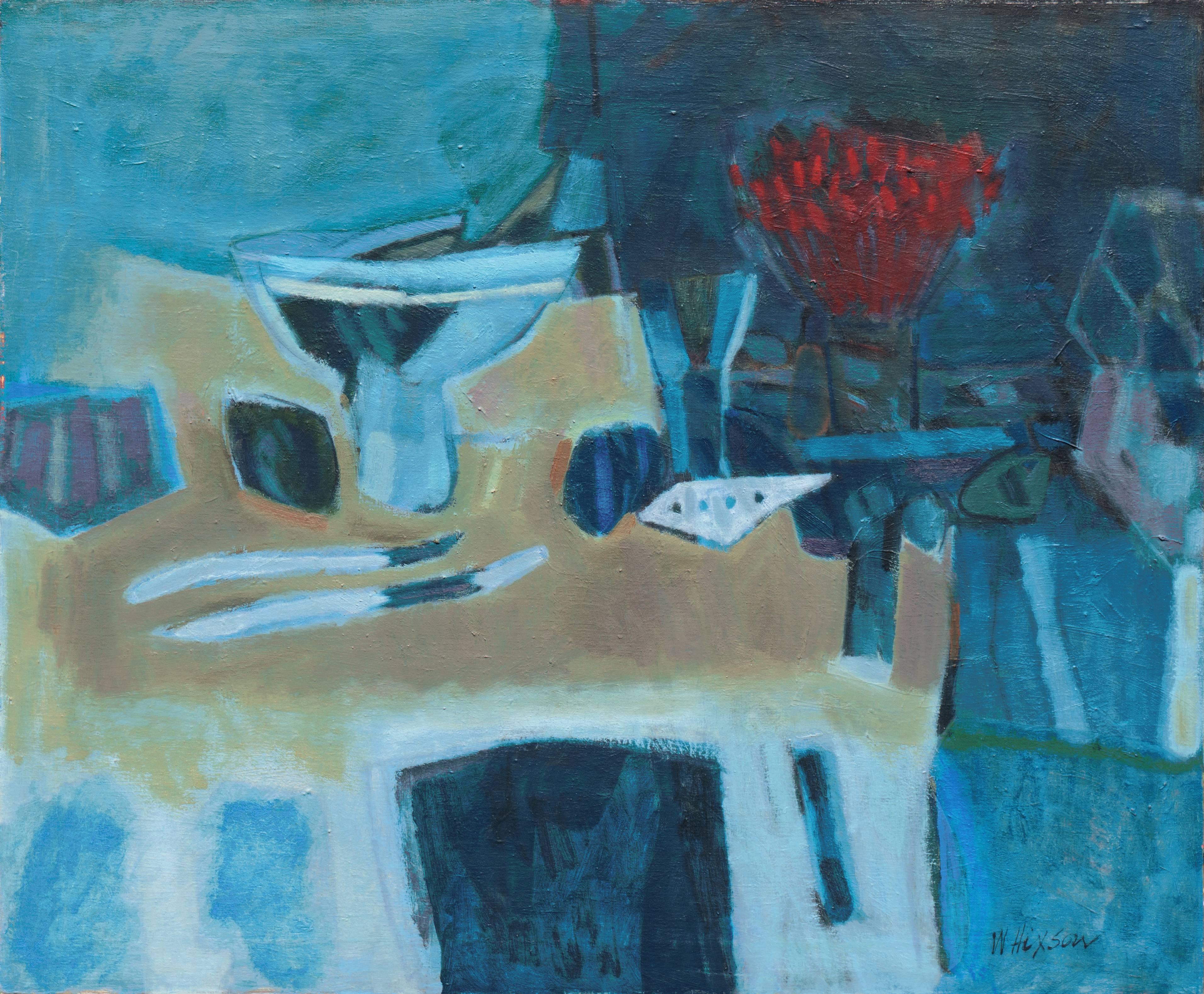This professionally done, modernist, rectangular painting predominantly showcases a geometric and slightly abstract scene set within a kitchen space, rendered in various shades of blue. The painting, possibly from the late 19th or early 20th century, captures a still life that’s reminiscent of cubist works like those of Picasso, yet signed in the bottom right corner by an artist whose name appears to be W-HEXSON or a variation thereof.

On the left side of the composition, there is a brown dining table, where the light brown sides and a slightly blurred brown top accentuate its presence. Central to the table is a footed bowl, light blue with a white trim, containing a couple of unidentifiable objects and accompanied by two long, silver knives laid out close to it. The details further suggest potential salt and pepper shakers, dark blue in color, and a glass placed to the right of the bowl. 

Amidst the various other parallelogram-shaped objects, a striped red and beige towel with a silvery border might be discernible to the left of the bowl. The upper left corner of the background remains light blue with visible paint textures, while the upper right corner shifts to a darker blue hue. Contrasting the surrounding blue tones is a vase placed prominently in the background, filled with very red flowers, possibly tulips, with unopened bulbs. Despite this abstract representation, the image vividly encapsulates a kitchen's dining area infused with modernist auras through an intricate play of colors, geometric patterns, and textures.